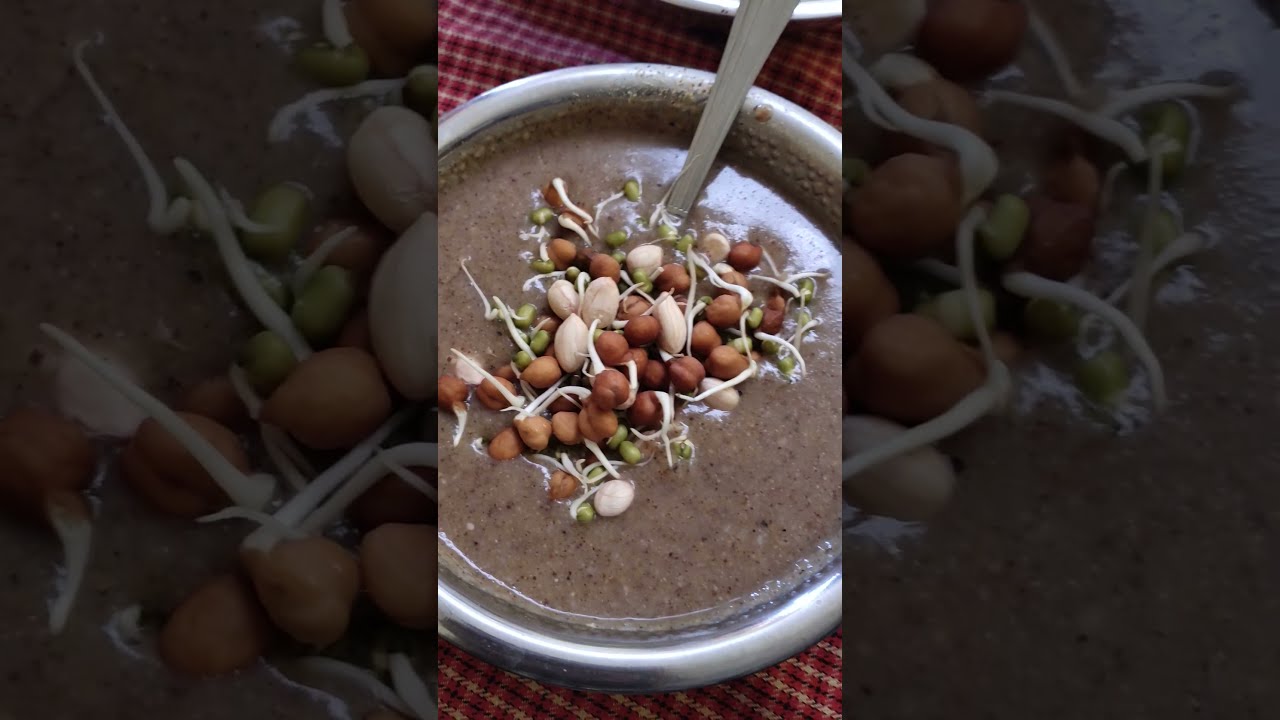The image features a composite layout with a central picture showcasing a white bowl filled with a brown, soupy liquid, and a mix of beans that are brown and light tan, possibly including green soybeans or edamame. Top of the dish appears to be garnished with a shredded white substance, which could be cheese or dough. A silver spoon is partially submerged in the bowl, positioned to stir the contents. The bowl rests on a red and white checkered tablecloth. The composition includes two magnified sections on the sides, focusing on the beans from the main image, but these are blurred and less colorful. The natural lighting of the setting suggests it was taken during daytime. The overall presentation is intricate and aesthetically appealing.